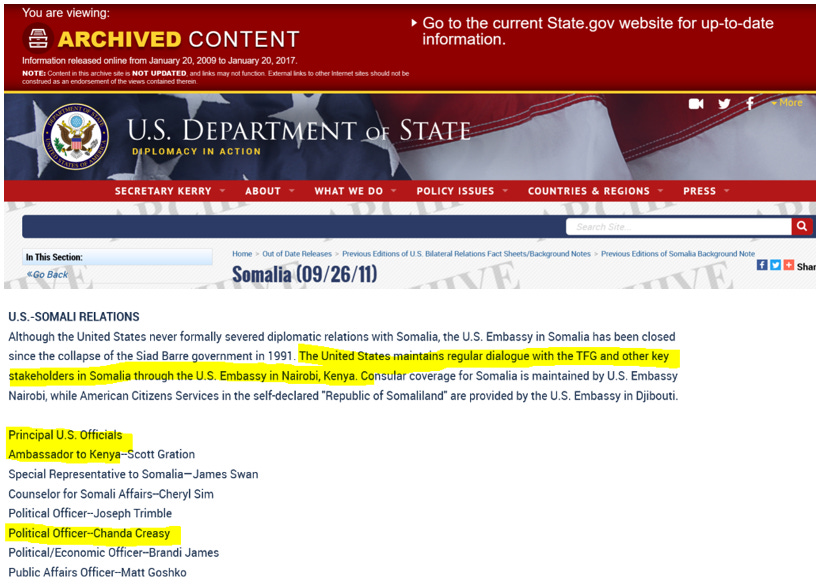In this image, a prominent red banner at the top indicates that the viewer is looking at archived content, featuring a file drawer icon. The banner reads, "You are viewing archived content. Go to the current state.gov website for up-to-date information." A white right arrow accompanies this message. Below, text specifies that the information was released online from January 20, 2009, to January 20, 2017, and has not been updated.

A yellow line separates the banner from the main content, which displays the seal of the US Department of State with the slogan "Diplomacy in Action." To the right of the seal, social media icons for Facebook and Twitter are visible.

Further down, a red block contains links to various sections including "Secretary Kerry," "About," "What We Do," "Policy Issues," "Countries & Regions," and "Press," each with small down arrows beside them.

A blue box follows, containing a white search bar and options labeled "In This Section" accompanied by a left arrow and "Go Back." Below this, there is text referencing "Somalia 092611" with a small blueprint above it. Social media icons for Facebook and Twitter appear again.

A section titled "US-Somalia Relations" is highlighted in yellow, stating, "The United States maintains regular dialogue with the TFG and other key stakeholders in Somalia through the US Embassy in Nairobi, Kenya." Alongside this, the text in yellow mentions "Principal US Officials," naming Ambassador to Kenya Scott Gration and Political Officer Chandra Creasy.